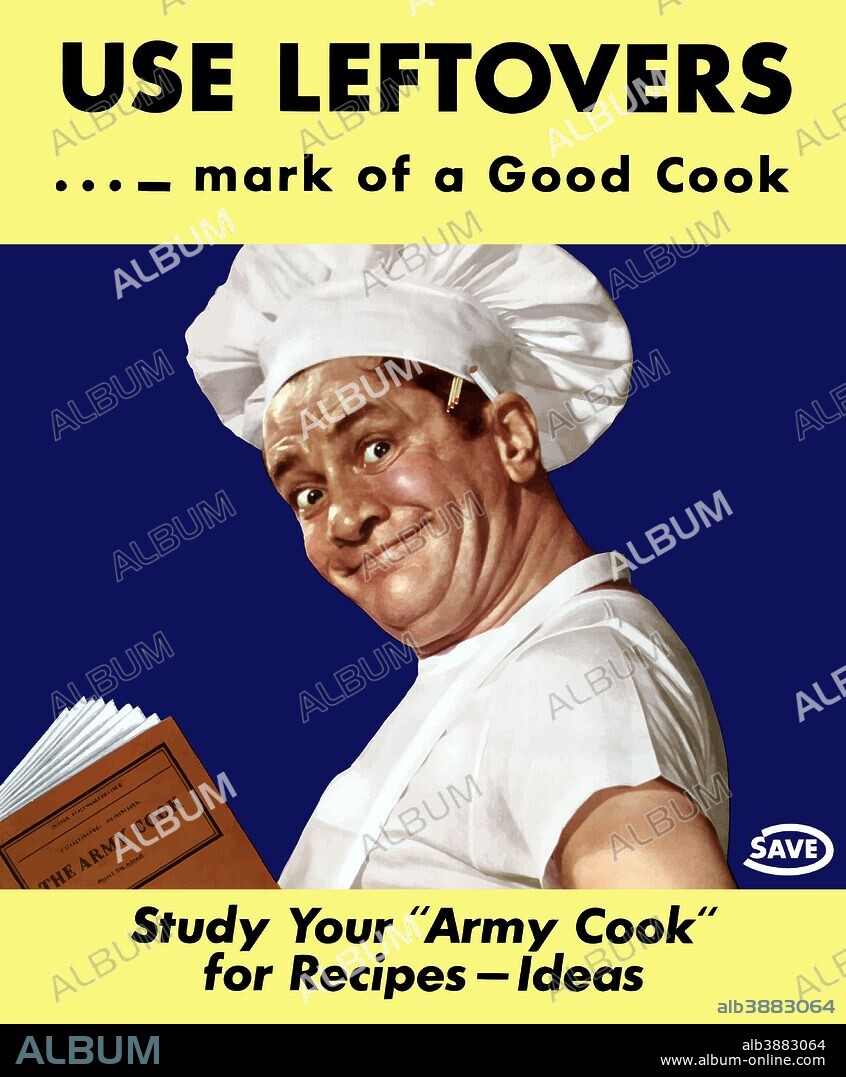This image is the cover of an old cookbook, prominently featuring a man in the center dressed in a full white chef's outfit, including a chef hat, apron, and t-shirt. The man holds a brown book titled "The Army Cook." He is smiling at the camera in an odd, toothless grin, with wooden matches clipped under his hat and a cigarette behind his ear. Behind him is a blue background, while the upper and lower sections of the cover are yellow. Bold black letters at the top read, "Use Leftovers.../ Mark of a Good Cook," and below the man's image, it says, "Study Your Army Cook for Recipes - Ideas." The bottom left corner of the cover contains the watermark "Album" from album-online.com, indicating the marketplace from which this stock photo originates.